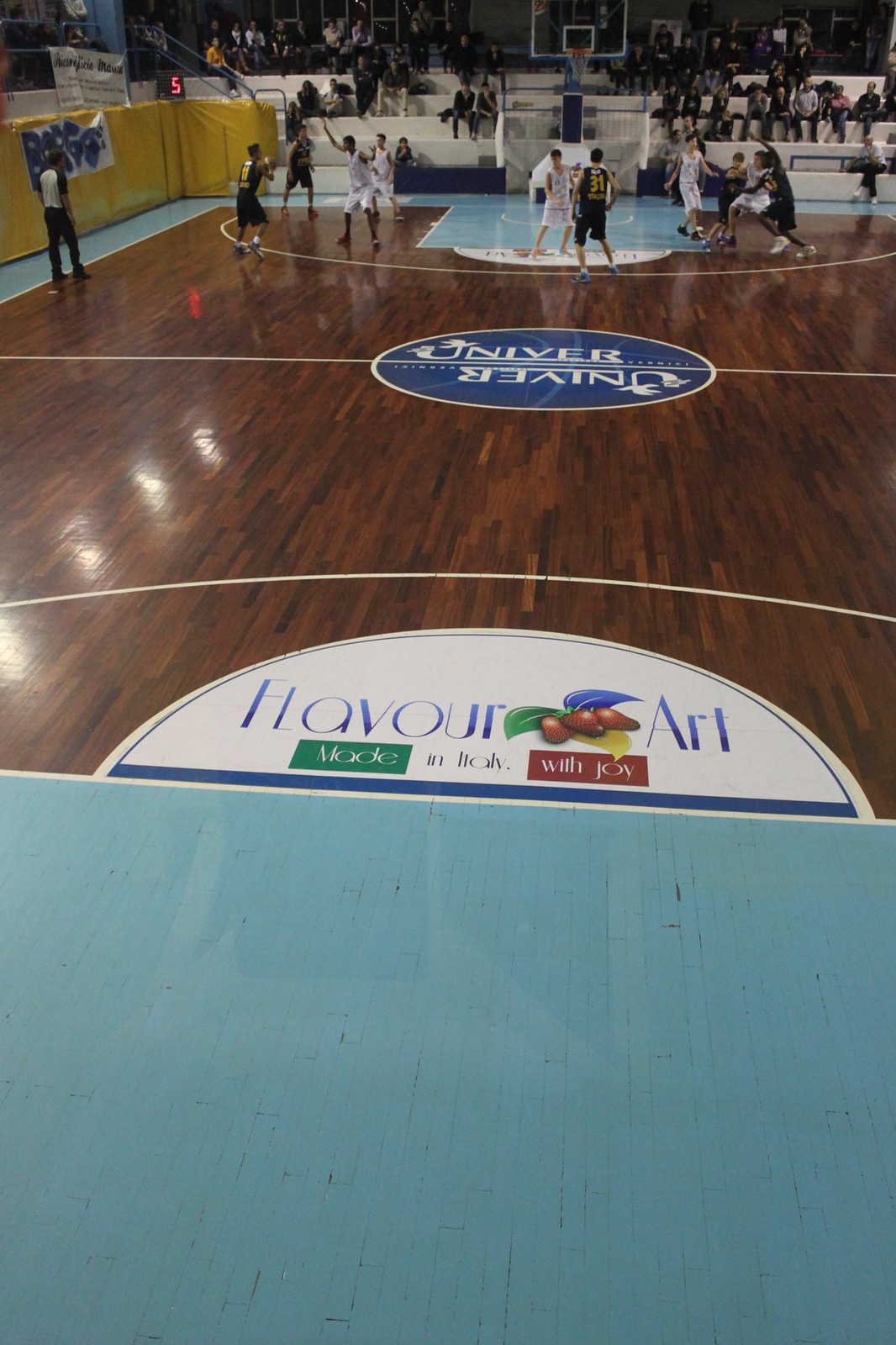This vertically aligned, colorful photograph captures a high school basketball game in session on a dark brown wooden court adorned with sponsor logos, notably "Havar Art made in Italy with joy." The scene features two teams of young players, one in predominantly black jerseys with yellow accents, and the other in white jerseys, engaged in gameplay near the basketball hoop. The action takes place in a gymnasium with a yellow wall and partially filled bleachers in the background. White lines crisscross the floor, marking the court boundaries and the circular center area. The bottom third of the image is obscured by a light blue tint, possibly part of the floor's design. A referee is visible on the sideline, overseeing the game, while the audience watches intently. No scoreboard is visible in the image.